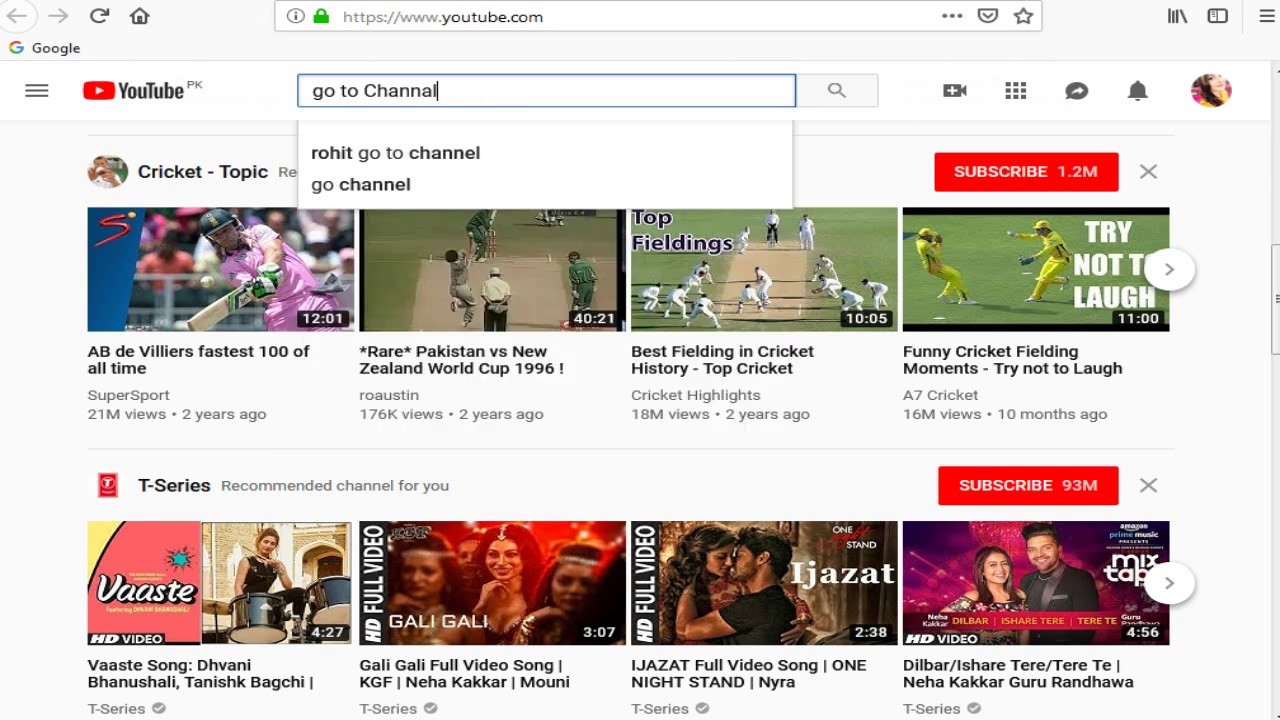The screen capture displays a YouTube webpage as seen on an Apple Mac device. The search bar at the top contains a slightly misspelled query, "go to Chanel," likely meant to be "go to Channel." To the right of the search bar are typical YouTube interface icons, including the upload button, notification bell, and the user's profile picture.

Below the search bar is a section titled "Cricket Topic" followed by four videos related to cricket. The first video is titled "AB de Villiers Fastest 100 of All Time." Adjacent to it is a video named "Rare Pakistan vs. New Zealand World Cup 1996." Next is a video titled "Best Fielding in Cricket History, Top Cricket," and the fourth video is "Funny Cricket Fielding Moments - Try Not to Laugh," which also displays a "Try Not to Laugh" banner on its thumbnail.

Beneath these videos, there is a recommended channel section prominently featuring the Indian music label T-Series. The recommended content includes titles largely in Hindi, such as "Vastisang Devani Benusali Tasikbagchi," "Golly Golly Full Video Song," "Izzazet One Night Stand," and "Dilbar I Share Tear Tear."